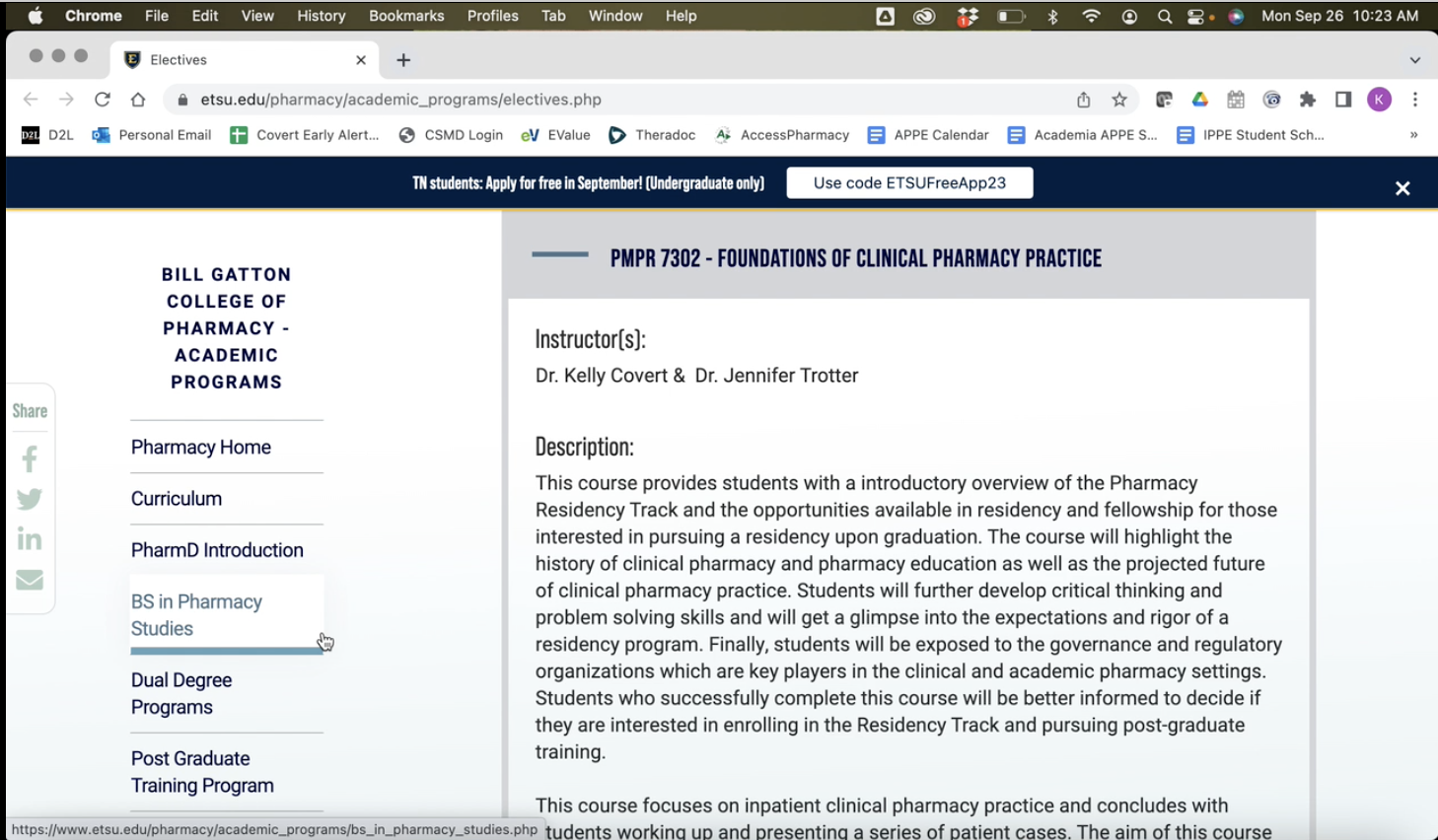This image is a detailed screenshot of a web page displayed in the Google Chrome browser on a Mac.

### Browser Details:
- **Browser**: Google Chrome, identifiable by the "Chrome" label on the top left and the white Apple icon to its left.
- **Active Tab**: The single open tab is gray and labeled "Electives."
- **Address Bar**: The URL shown is `etsu.edu/pharmacy/academic_programs/electives.php`.
- **Top Border**: The browser's top border is black, displaying date and time information on the right side, indicating "Monday, September 26, 10:23 a.m."

### Web Page Details:
- **Banner**: A dark blue, narrow banner at the top features important information in white font: "TN students apply for free in September (undergrad only)." A white rectangle within this banner states: "Use code ETSUFREEAPP23."
- **Sidebar**: 
  - The background is white with a left-hand sidebar.
  - Sidebar Header: "Bill Gatton College of Pharmacy Academic Programs."
  - Sidebar Items:
    - Pharmacy Home
    - Curriculum
    - Pharm D Introduction
    - BS in Pharmacy Studies
    - Dual Degree Programs
    - Postgraduate Training Programs

### Main Content:
- **Course Title**: Centered on the right side of the page, the course title "PMPR 7302 Foundations of Clinical Pharmacy Practice" is displayed in dark navy blue font against a gray background.
- **Course Information**:
  - Below the title, the section shifts to a white background with dark gray font.
  - **Instructors**: Dr. Kelly Covert and Dr. Jennifer Trotter.
  - **Description Heading**: The word "Description" precedes a paragraph of detailed text about the course.
- **Additional Information**: Beneath the description paragraph, the first two lines of the following section are partially visible, suggesting more detailed course content or prerequisites might follow.

Overall, the screenshot provides a comprehensive view of a specific course page within the East Tennessee State University (ETSU) Pharmacy academic program listings.